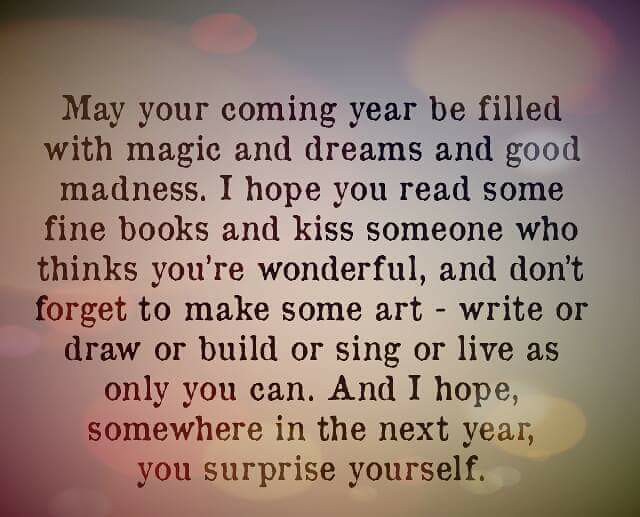The image features a motivational quote in black machine-printed text against a light-colored background adorned with faint, circular patterns resembling bubbles in hues of red, green, blue, and yellow. The paper has a subtle glare, particularly at the corners, adding a slightly darker contrast. The quote reads:

"May your coming year be filled with magic and dreams and good madness. I hope you read some fine books and kiss someone who thinks you're wonderful. And don't forget to make some art—write or draw or build or sing or live as only you can. And I hope somewhere in the next year you surprise yourself."

This descriptive, detailed caption combines elements of the bubble-like colorful background and emphasizes the motivational message of the card.